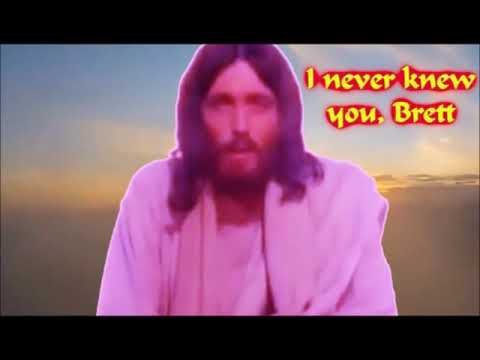The image features a grainy and slightly blurred depiction of a stereotypical Jesus figure against a dreamlike sky-scape. Jesus, a white male with shoulder-length, slightly curling hair, is dressed in white or whitish-brown robes, although the entire scene is cast in a pinkish-purple hue. The background consists of a surreal, nebulous sky with wispy yellow clouds blending into a blue expanse. Jesus' image emanates a soft glow and appears somewhat translucent. Black horizontal bands frame the top and bottom of the picture. On the upper right side, in stylized gold text with red shadows, it reads, "I never knew you, Brett," lending a mysterious and somewhat eerie tone to the scene.